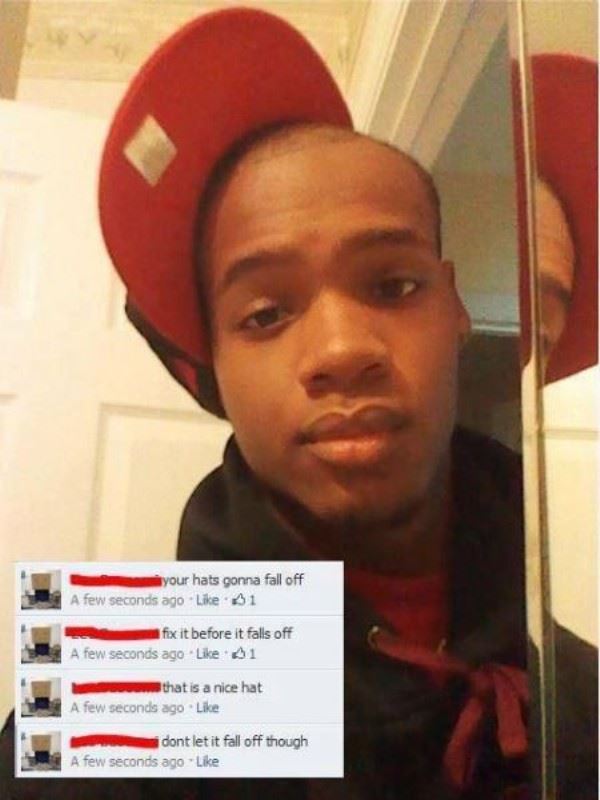The photograph depicts a young African-American man standing in a doorway, likely of his bathroom, with a beige ceiling and a white door visible in the background. He is dressed in a black hoodie adorned with red strings and a red baseball cap perched sideways on his head, with the bill also red. A mirror on the right side of the image captures a partial reflection of him, and his serious expression suggests a candid moment. The bottom left corner of the picture contains various social media comments on a white background. The comments predominantly mention the precarious position of his hat, urging him to fix it before it falls off. Specifically, the comments read: "Your hat is going to fall off," "Fix it before it falls off," "That is a nice hat," and "Don't let it fall off though." The colors in the image include whites, off-whites, yellows, reds, and blacks. Overall, the setting, the reflections, and the casual stance suggest this is a social media post capturing a moment of spontaneous fashion and interaction.